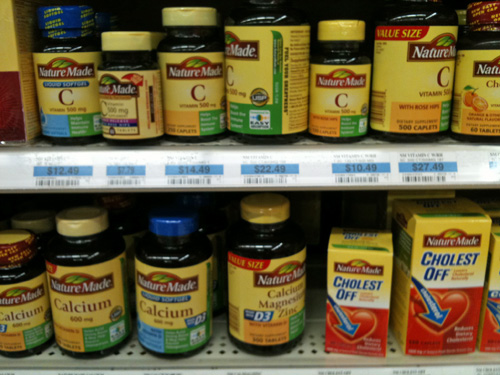The image features two shelves filled with various supplement containers. 

On the bottom shelf, there are five bottles of calcium supplements. Four of these bottles have yellow lids, while one has a blue lid. Alongside these, there are several containers of magnesium and CholestOff supplements. CholestOff is represented by both a small and a large box.

The top shelf has multiple price tags, showing amounts like $12.49, $7.75, $14.49, $22.49, $10.49, $27.90, and $27.49. This shelf holds several "Nature Made" brand supplements, all labeled with the letter "C." They are stored in bottles with yellow lids, except for the one on the far left, which has a blue lid adorned with yellow writing.